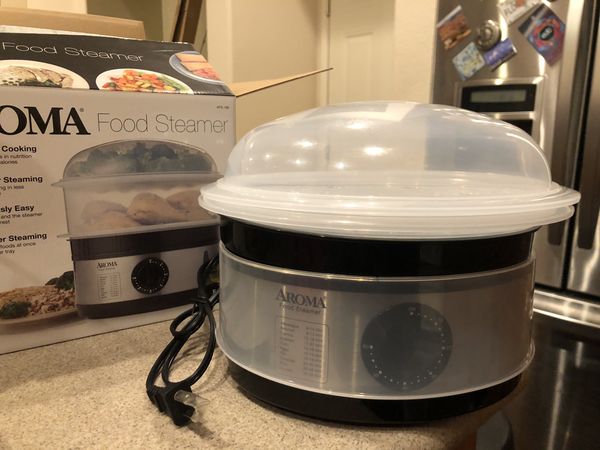The image showcases a recently unpacked Aroma food steamer positioned prominently on a kitchen counter. The steamer itself is located in the bottom right of the image, featuring a slightly translucent white plastic cover resembling Tupperware, and a black dial-coated base, also wrapped in protective plastic not seen on the packaging. The product's name, “Aroma,” is clearly visible on both the steamer and its box, which sits to the left. The box displays an image of the food steamer along with partially obscured text hinting at ease of use in cooking and steaming. The kitchen setting is further detailed by a stainless steel refrigerator with a digital interface to the right, adorned with various postcards or pictures held up by magnets. Colored accents in the image include black, white, silver, red, orange, green, purple, and blue, adding vibrancy to the scene. A black cord is also visible to the left of the steamer, enhancing the freshly unpacked feel.